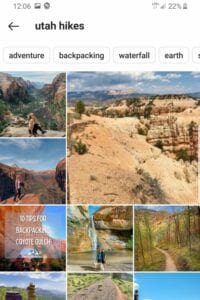A screenshot depicting a phone search for "Utah Hikes" is shown on a white background. At the top-left corner of the screen is the time displayed as "12:06," followed by a small picture icon and a circular icon. On the far-right corner, there is a connectivity bar, the text "22%" indicating battery life, and a battery icon. Directly below this information is a back arrow to the left and black text that reads "Utah Hikes."

Beneath the main header are four text bubbles with the labels "Adventure and Backpacking," "Waterfall," and "Earth," respectively. Below these are several images showcasing various canyons and hiking spots in Utah. On the left side, there are three vertically aligned, partially square images displaying rocky canyons with predominant shades of brown and burnt umber, contrasted with bright blue skies and white clouds, alongside some scrub brush. To the right, there is a larger picture of an expansive canyon landscape featuring scattered evergreens and scrub trees over weathered terrain.